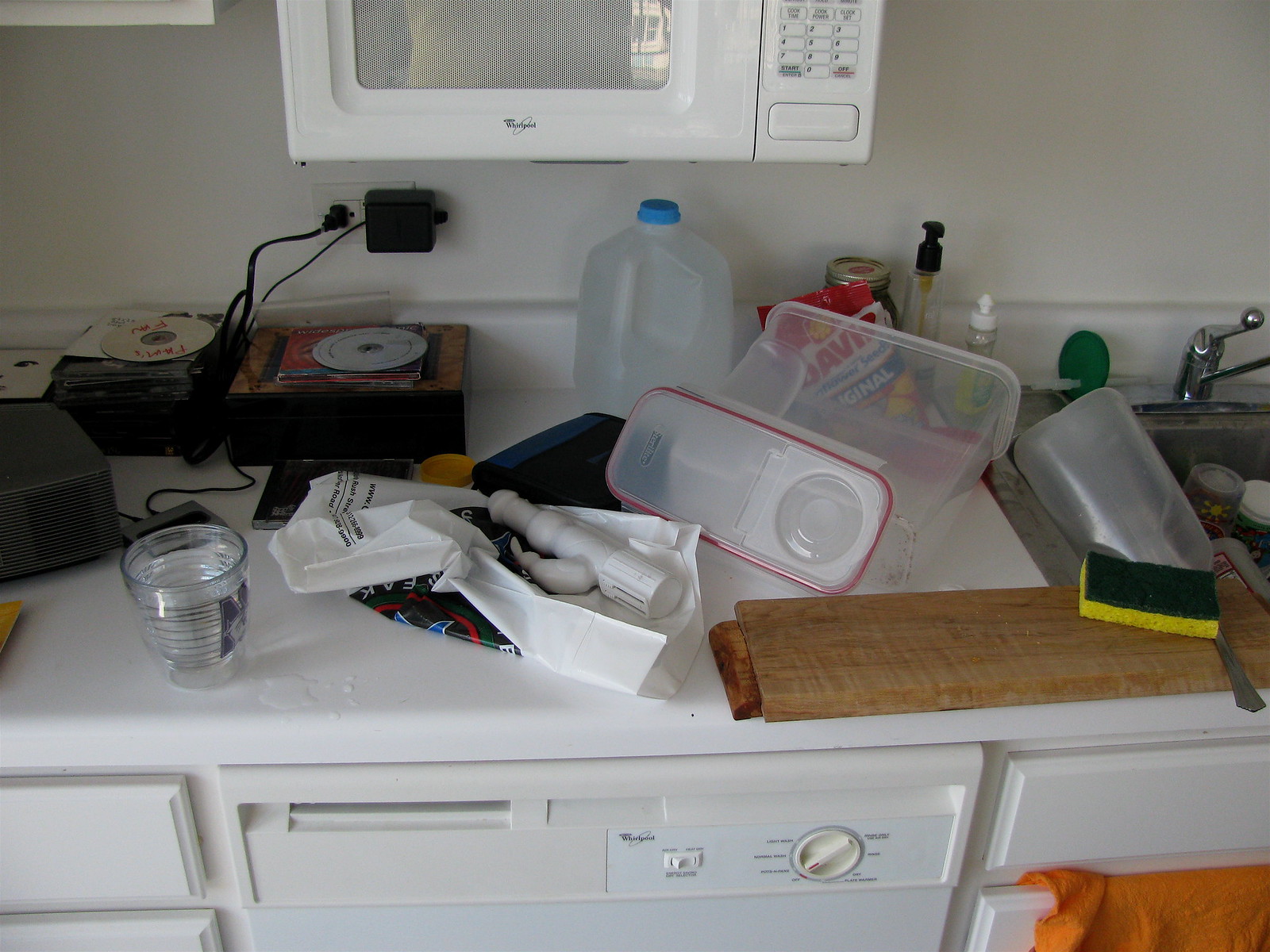This image features a small, compact galley kitchen typical of an apartment, showcasing a white linoleum countertop that extends into view. The upper portion of a white dishwasher is visible beneath the counter. The lower cabinets and drawers, also white, are partially shown, with a drop-down microwave peeking out from the top set of cupboards. The wall behind these features is similarly white, adding to the kitchen's clean and bright aesthetic.

On the countertop, there is a cereal saver—a plastic container designed for cereal storage. A water-filled milk jug and an unusual stack of CDs are also present, adding a touch of randomness to the scene. Nearby, some crumpled up paper, possibly instructions or notes, are scattered around.

To the right, the edge of the sink is visible, containing a yellow sponge with a green scrubby side facing up. Inside the sink appears to be another pitcher. Behind the sink is a package of David’s sunflower seeds, identifiable by the red and white packaging. Additionally, a retainer case is situated near the sink handle, adding a personal touch to the otherwise typical kitchen environment.

While the sink contains more items, they remain indistinguishable in the current view. The overall impression is of a small but functional kitchen filled with everyday items.